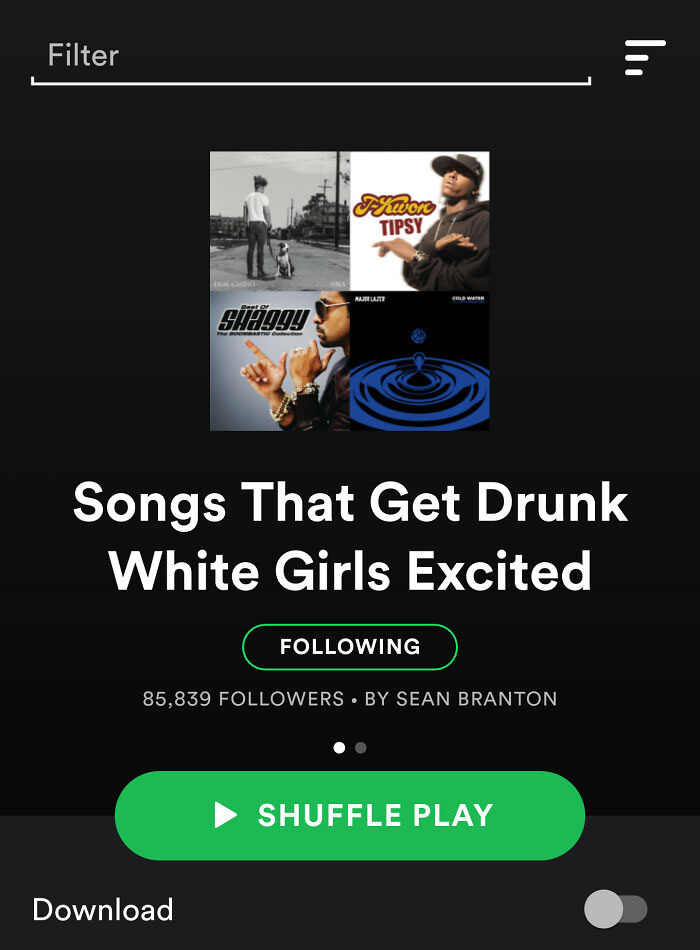This image appears to be a screenshot from a music streaming website or app with a black background and a vertical rectangular shape. 

**Top Section:**
- *Top Left*: The word "Filter" is displayed in light gray letters.
- *Below Filter*: A thin white horizontal line.
- *Top Right*: There are three horizontal bars, placed one above the other, indicating a menu icon.

**Middle Section:**
- *Center*: A large square is present, divided into four smaller segments, each featuring an album cover.
  - *Top Left Segment*: Displays a black and white photo of the back of a man walking a dog on a leash.
  - *Top Right Segment*: Shows an album cover with text that appears to include the word "Tipsy" and features a guy in a black cap and black hoodie.
  - *Bottom Left Segment*: Contains the text "Shaggy," with a side profile image of a man pointing with one finger and resting his chin on his other hand.
  - *Bottom Right Segment*: Displays an album cover that is difficult to read, featuring a black background with blue water drop imagery.

**Below the Square:**
- In white text, it reads: "Songs that get drunk white girls excited."
- An area labeled "Following" is present, indicating the playlist has 85,839 followers and is curated by Sean Branton.
- A large "Shuffle Play" button is located below this information.
- At the very bottom, there is an option to "Download."